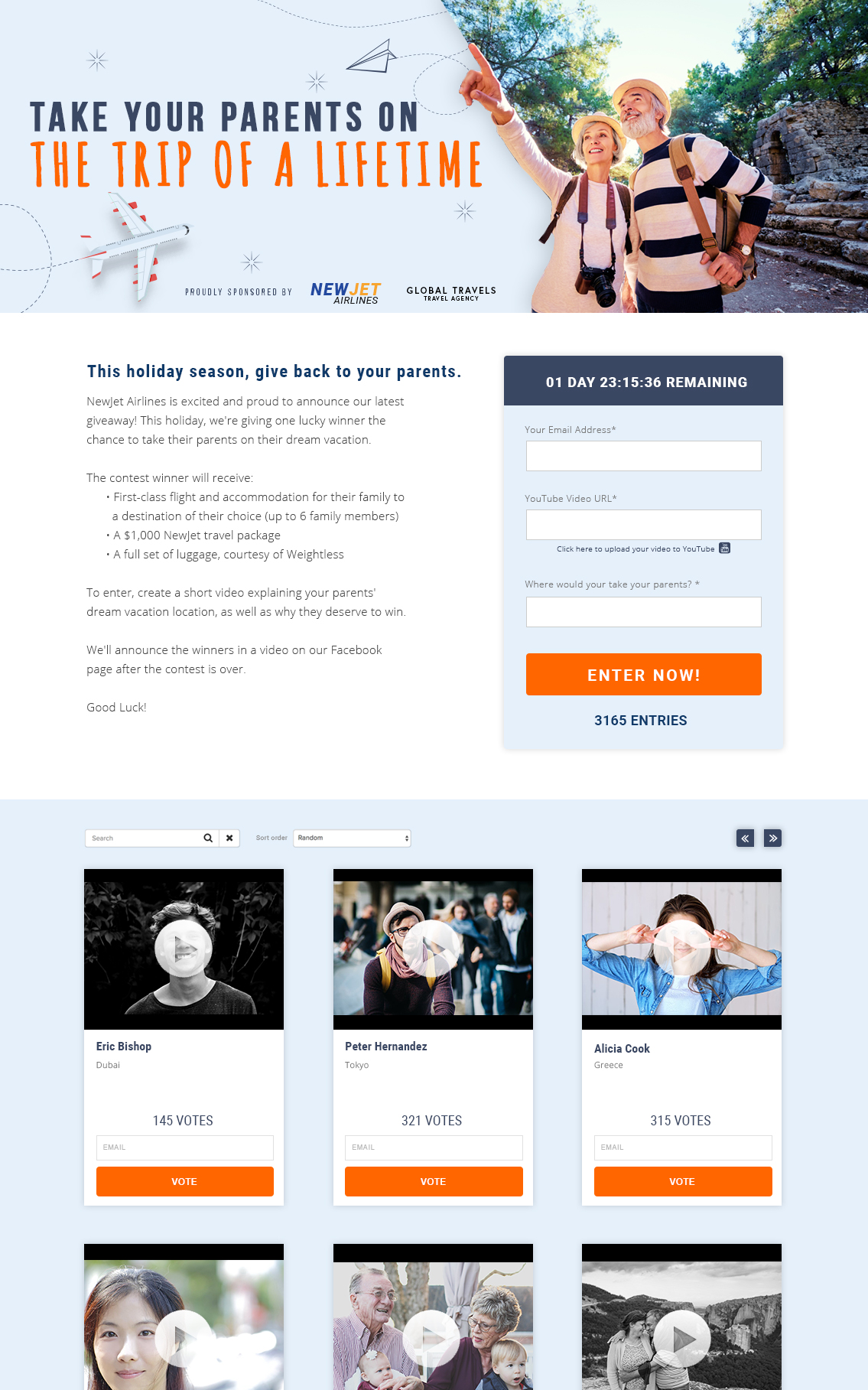**Signup Page for "Take Your Parents on the Trip of a Lifetime" Sweepstakes**

The top third of the signup page features the headline: **"Take Your Parents on the Trip of a Lifetime."** The phrase "Take your parents on" is rendered in a dark blue or almost dark gray, while "the trip of a lifetime" stands out in an eye-catching playful orange font. Immediately below this heading, there's a captivating bird's eye view of a jet plane executing a loop-de-loop.

The background against this scene is a soothing blend of light gray and very light blue, seamlessly transitioning to an image on the right. This image showcases an elderly couple: the woman is raising her right hand, pointing towards the sky, and the man, wearing a hat and a brown backpack strap over his shoulder, looks up in the same direction. Behind them, a picturesque natural setting unfolds with trees, a bright sky, and striking ancient stone steps to their right.

The middle portion of the page, taking up about a third of the layout, has a white background. On the left side, the text reads: **"This holiday season, give back to your parents"** in blue, followed by some plain text descriptions underneath. To the right, a sign-up box is prominently displayed, showing a countdown timer with **"1 day 23 hours 15 minutes and 33 seconds remaining."** There are three text boxes for users to input their information: **Email Address** (required), **YouTube Video URL** (required), and **Where You Would Like to Take Your Parents** (required). An orange **"Enter Now!"** button with white font encourages users to submit their information. Below this button, there is a line of blue text stating: **"3,165 entries"**.

At the bottom of the page is a section with a blue background, offering users the chance to vote for different videos. This grid layout displays three columns of video uploads. Each video thumbnail has a stock image, potentially depicting a person or a couple, with an orange **"Vote"** button at the bottom. Above each button, the number of votes is shown. The videos feature:
- Eric Bishop from Dubai with 145 votes
- Peter Hernandez from Tokyo with 321 votes
- Alicia Cook from Greece with 315 votes

There are three additional video thumbnails partially visible beneath these, but their vote counts are not displayed.